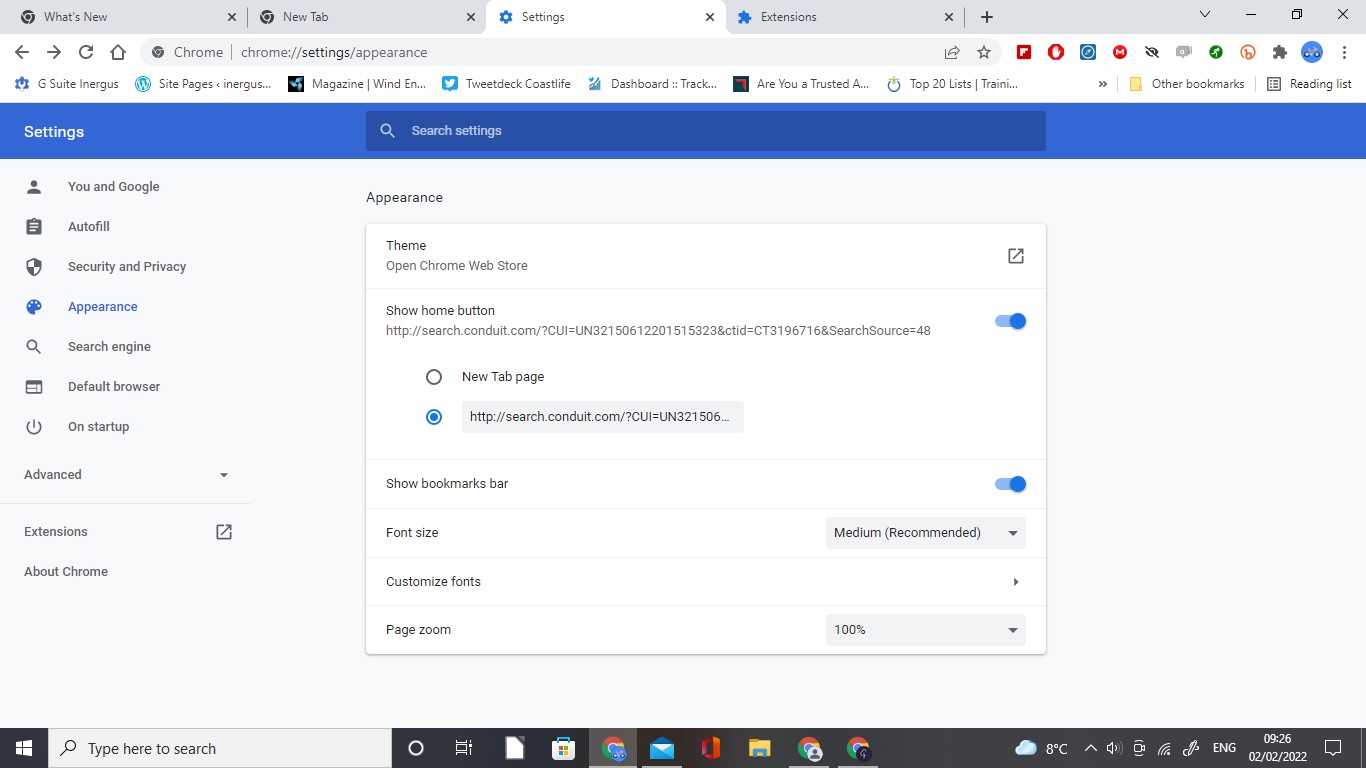This image is a detailed screenshot taken in landscape mode, depicting the "Appearance" settings page of Google Chrome. 

In the upper left corner, there is a row of tabs in a gray-colored bar. From left to right, the tabs are labeled: "What's new," "New tab," and in white, "Settings." The row then continues in gray with "Extensions" and an option to add a new one. 

The next row displays Google Chrome's settings sections, prominently highlighting the "Appearance" tab in blue along with a search bar labeled "Search settings." On the left-hand side of the screen, a navigation panel lists various setting categories: "You and Google," "Autofill," "Security and privacy." The "Appearance" tab is highlighted in blue, indicating the active section, while other categories listed include "Search engine," "Default browser," "On startup," "Advanced," "Extensions," and "About Chrome."

On the right side, under the "Appearance" settings, there's a white form interface. It starts with the "Theme" section, offering a link to "Open Chrome Web Store" for theme options. The next section is "Show home button," which includes a text field for the home button URL and a toggle switch turned on. Users can select between a new tab page or a custom URL, such as "search.conduit.com," for the home button.

Following that, the option "Show bookmarks bar" has its toggle switch enabled. The "Font size" setting is set to "Medium" as recommended, with an option to customize fonts if preferred. Finally, "Page zoom" is configured at 100%, denoting standard display zoom.

This comprehensive screenshot provides a clear and detailed view of the various customizable appearance settings within Google Chrome.